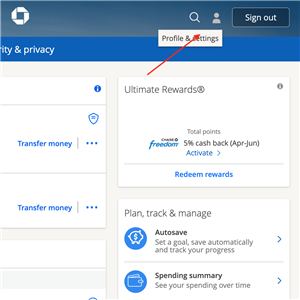The image captures a user interface on a smartphone screen, likely showing a financial management or rewards program application. At the top of the screen, there is a navy-blue bar with white text reading "Sign Out," along with an emblem, a search icon, and a person icon. Below this bar, partially visible text seems to read "urity and privacy," suggesting "Security and Privacy."

Prominently, a digitally added red arrow points toward the "Profile Settings" section. The screen displays multiple interactive features:

- **Transfer Money:** Appearing twice with a protective shield icon.
- **Ultimate Rewards:** Featuring a summary titled "Total Points."
- **Chase Freedom 5% Cash Back April through June:** Accompanied by an "Activate" button.
- **Redeem Rewards:** For utilizing accumulated points.
- **Plan, Track, and Manage:** Sections for organizing financial activities.
- **Auto Save:** Indicated by a piggy bank icon with a dollar sign.
- **Spending Summary:** Identified by a wallet icon within a blue circle.

The interface suggests a comprehensive digital tool for managing finances, rewards, and savings, providing users with detailed information and actionable options for their financial activities.